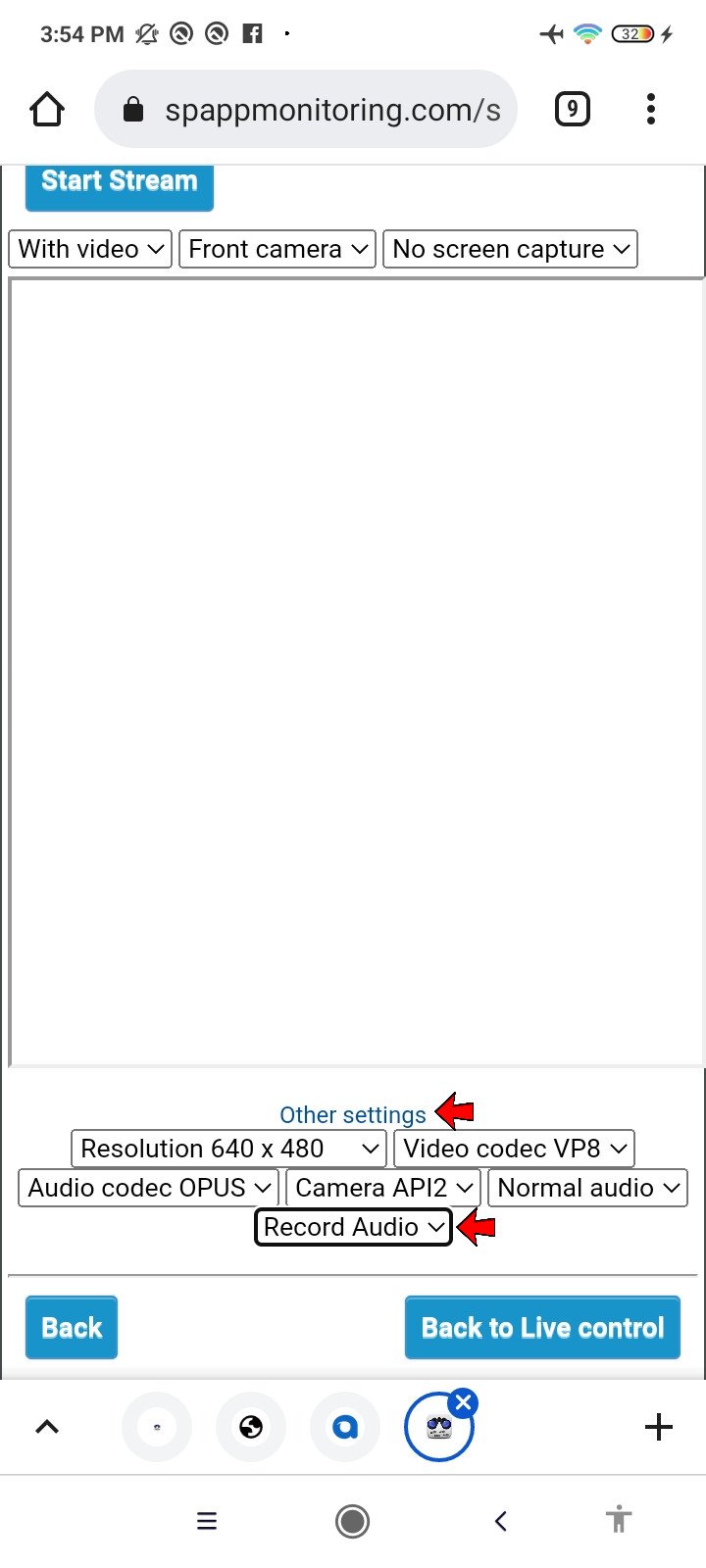A detailed screenshot of a smartphone screen taken at 3:54 PM. The phone, currently in airplane mode, shows a battery level of 32%. At the top, multiple icons are visible, including the Facebook icon. The screen indicates it’s on a secure site, displaying "spappmonitoring.com".

Below the URL, on the upper left, a blue button labeled "Start Stream" is visible. Adjacent to the button, options for “Video,” “Front Camera”, and “No Screen Capture” are displayed. The majority of the screen is empty, with a large white blank area.

Further down, centered and clickable blue text with settings options is highlighted by a thick red arrow pointing towards it. Directly beneath, two stacked boxes provide settings for "Resolution: 640 x 480" and "Video Codec: VP8," both with dropdown menus. In the middle section, additional dropdown settings for "Audio Codec: Opus," "Camera API: 2," and "Normal Audio" are available.

Toward the bottom, a red arrow points to the "Record Audio" option featuring a dropdown menu. Finally, at the very bottom of the screen, two buttons are visible: one labeled "Back" on the left and the other "Back to Live Control" on the right.